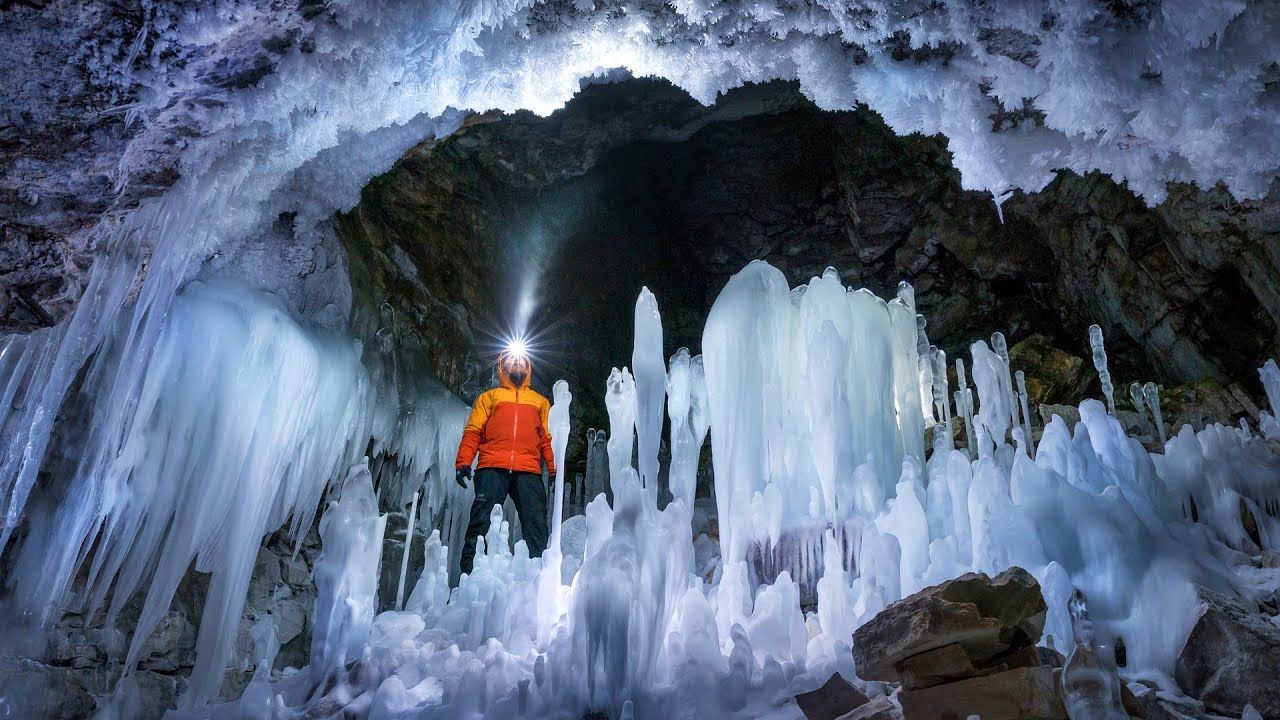In this captivating photograph taken inside an underground cave, an explorer dons a bright orange and yellow puffy winter jacket with a hood, paired with black ski pants or possibly blue jeans. The explorer is equipped with a headlamp, which is the sole light source in the otherwise dark environment. This headlamp casts a glow upwards, illuminating both the top of the cave and numerous icicles that stretch from the ceiling. The cave's ceiling and floor are adorned with impressive formations of white ice, including long, tall icicles rising from the ground and shorter, sharper ones hanging from above. The surrounding rock walls are predominantly gray with black sections, adding contrast to the icy spectacle. Scattered boulders add rugged texture to this stunning subterranean landscape.